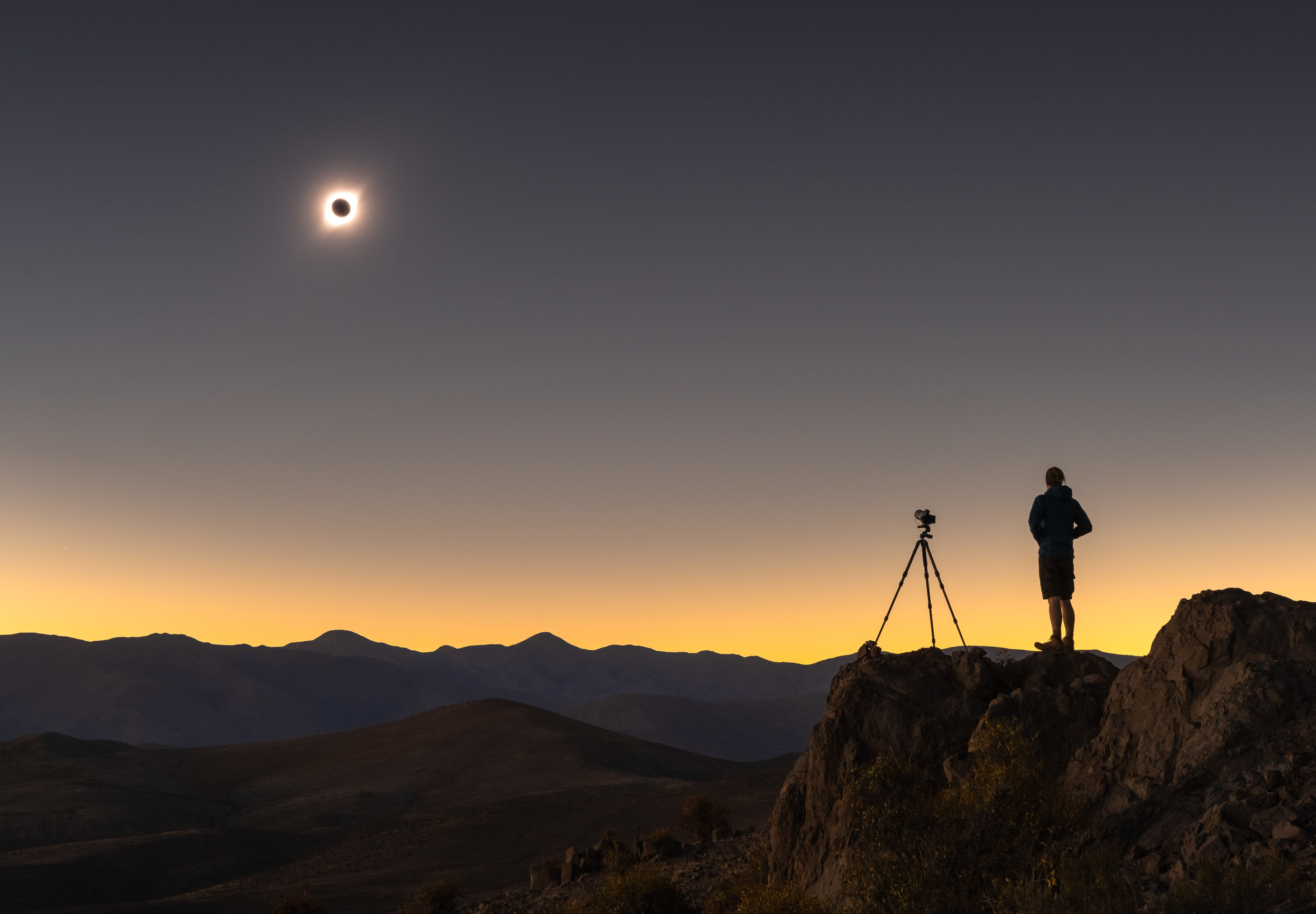In this stunning landscape photograph taken during a solar eclipse, a man stands in the lower right-hand corner, poised with either a camera or telescope on a tripod. With his back to the viewer, he gazes up at the dramatic celestial event. The eclipse dominates the upper left quadrant of the image, with the moon perfectly aligning in front of the sun, creating a glowing corona effect that illuminates the darkened scene. The setting appears to be a rocky, desert-like environment reminiscent of Arizona or Colorado, featuring brown mountainous terrain. The sky is layered, with a gray expanse covering the upper half, transitioning through bands of pinkish-gray and warm yellow light near the horizon, casting a subtle glow over the rugged landscape. The overall atmosphere is serene and hauntingly beautiful, marked by the profound stillness of the eclipse's twilight.